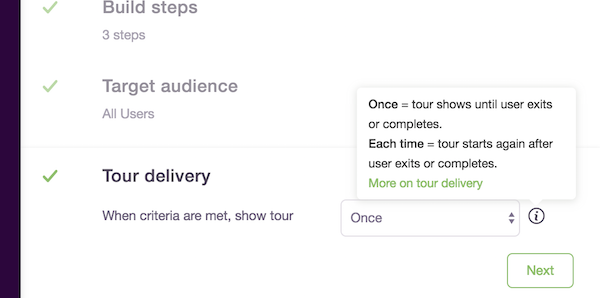This image is a detailed process flowchart, landscape in orientation and rectangular in shape, with a prominent purple vertical bar along the left edge. The purple bar is slender yet tall, stretching approximately eight times its width.

The chart outlines three specific steps, each accompanied by a green checkmark to the left. Though the first two steps are grayed out, the third one is highlighted, signifying the current focus. The steps proceed as follows:

1. **Build Steps**: Marked with a green checkmark, this section is labeled "Build Steps" and mentions "three steps" underneath.
2. **Target Audience**: Also marked with a green checkmark, this step specifies the audience as "All Users."
3. **Tour Delivery**: The highlighted and most detailed section, it states "When criteria are met, show tour." A white box to the right provides further clarification in black text: 
    - "Once equal, tour shows until user exit or completes."
    - "Each time equal, tour starts again after user exit or completes."
   Below this text, the phrase "More on tour delivery" appears in green.

Beneath the textual instructions, there is an additional white rectangular box labeled "Once," with options to add or subtract from it. A green "Next" button is positioned below this box, indicating the path to proceed in the process.